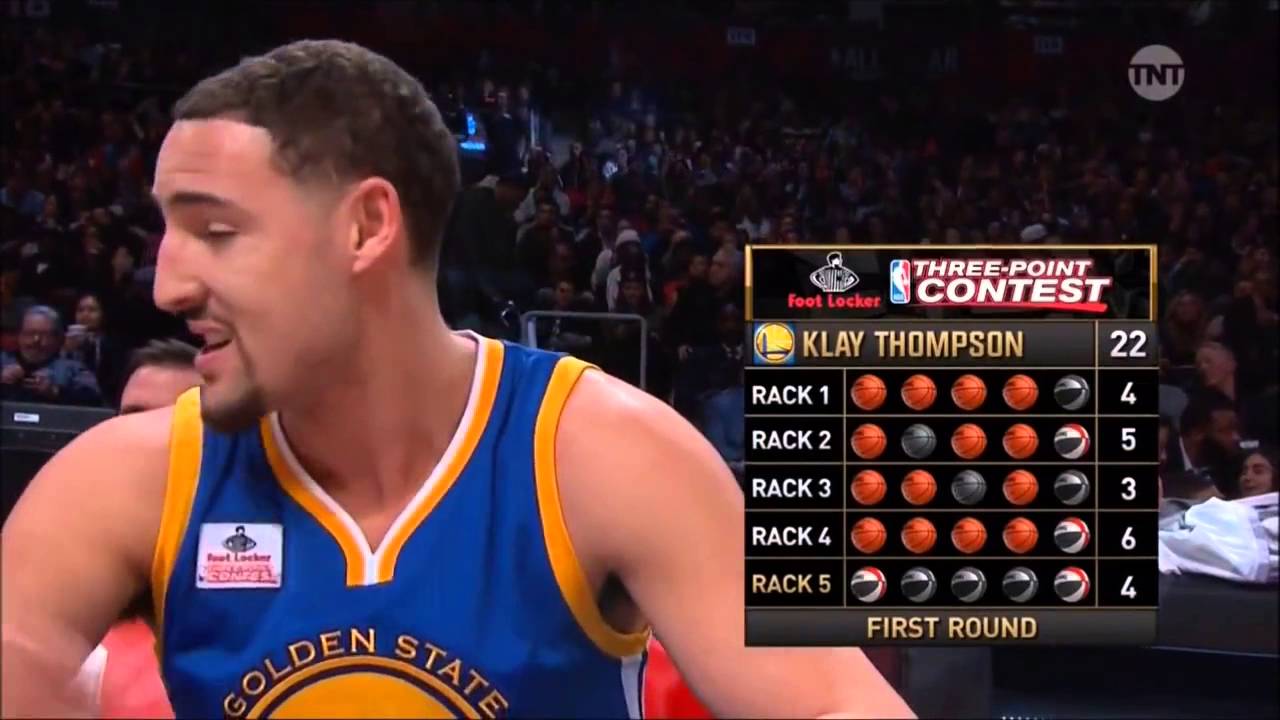The image is a screenshot from a TNT broadcast of a basketball event, specifically the Foot Locker Three-Point Contest featuring Klay Thompson. In the foreground on the left, a basketball player with a slightly mixed race complexion, short shaved black hair with a slight curl, and a goatee is looking to the left. He is wearing a blue sleeveless Golden State Warriors jersey with yellow and white trim, displaying "Golden State" in gold arching text across the chest and a visible white badge with a black logo and red text. 

In the background, the crowd is blurred and indistinct. On the right side of the image, there's a scoreboard graphic that includes vital details: the NBA logo, "Three Point Contest" text, Klay Thompson's name, followed by "Rack 1, Rack 2, Rack 3, Rack 4, Rack 5" each listed with their respective scores of 4, 5, 3, 6, and 4. His total score of 22 is prominently displayed. The bottom of the graphic reads "First Round" in yellow text, and it is visible that Thompson’s jersey has a small tag seeming to say "Red Lobster" alongside the Foot Locker logo.